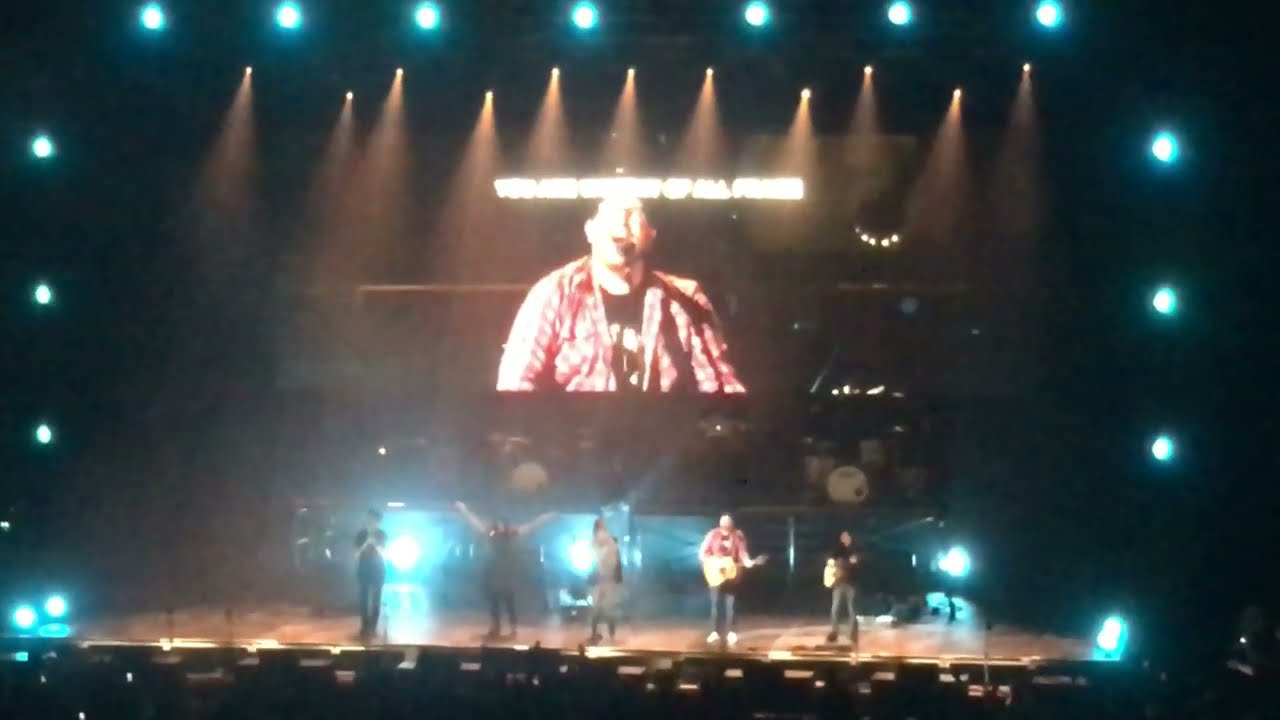The image depicts a nighttime concert scene with a lively band performing on stage. Dominating the top center of the image is a large screen displaying a close-up of one of the performers, who is wearing a red button-down shirt over a darker undershirt and a hat. The stage is set against a predominantly black background, illuminated by bright neon blue lights that appear as circular patterns around the stage. The performers, holding guitars and other instruments, are surrounded by an array of colors including brown, yellow, light blue, tan, white, orange, pink, and purple. The scene is vibrant and dynamic, suggesting an engaging live performance. No text is visible in the image.